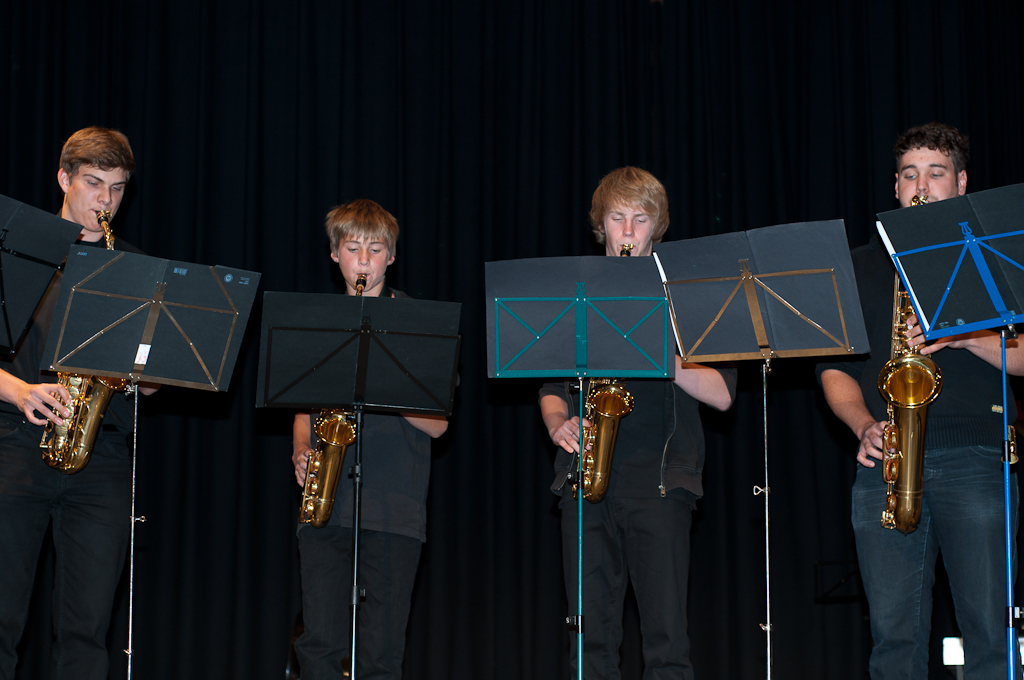The image is a color photograph depicting a youthful band of four boys, seemingly between 19 to 22 years old, each playing a saxophone. The boys are performing on a stage, standing behind music stands of varying colors, including brown, black, aqua, and blue. Each stand holds a black music book facing the players. They are uniformly dressed in black T-shirts, with three wearing jeans of different shades and one also sporting a jacket. The saxophones they are playing are bright and golden. Three of the boys, standing from the left to the center-right, have blonde hair, while the boy on the far right has black curly hair. The backdrop features a dark curtain, framing the stage. There is an even spacing between the boys, who appear to be intently focused on their music sheets as they play. Three of them are Caucasian, while one appears to be Mexican, adding a touch of diversity to the scene.